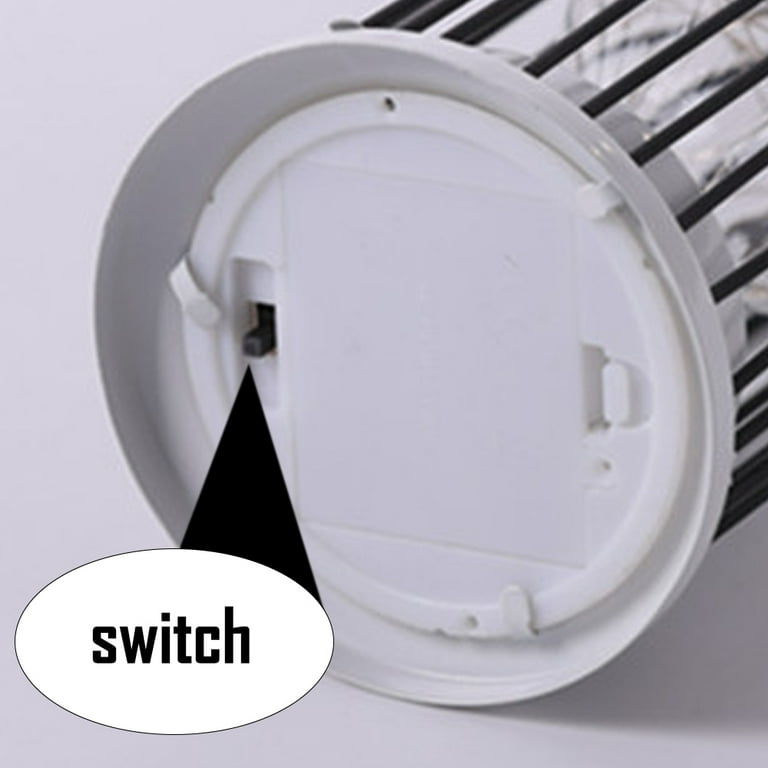This black-and-white photograph captures the bottom of an undetermined electronic instrument, showcasing a predominantly white plastic base. Centrally featured is a circular section that appears to be the access point for the battery compartment, complete with a latch mechanism for easy opening. Surrounding this circular base are three supporting pegs, ensuring stability when the device stands upright. Prominently displayed is a black switch in the down position, with an adjacent black triangle indicating its direction. Notably, a printed label, reading "switch" in large, lowercase black letters, points directly to this switch. Additionally, a black lever on the right side seems to facilitate access to the aforementioned battery compartment. This detailed and descriptive image likely serves as a guide for users needing to interact with the switch and battery compartment of the device.